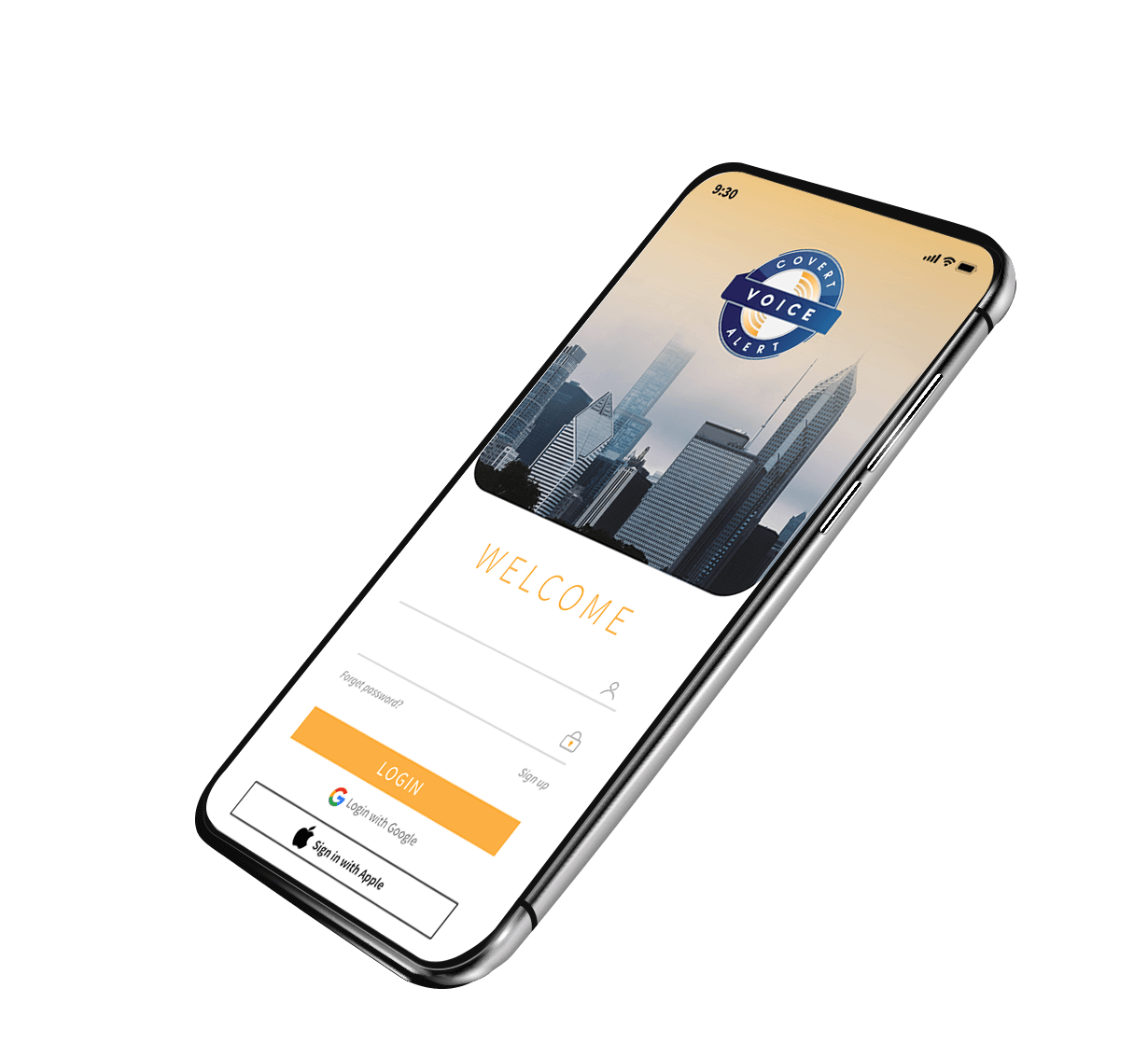The image showcases a sleek cell phone displayed against a white background, viewed at a slight angle. The phone screen is visible, with the bottom right corner positioned towards the bottom left of the frame and the top right corner aligned with the top right of the frame. The screen displays the time as 5:30, along with signal, Wi-Fi, and battery icons.

Prominently featured on the screen is a blue circle with the text "COVERT" inside it. Superimposed on this circle is a blue banner with the word "VOICE" in white, and "ALERT" is displayed at the bottom within the circle, forming the phrase "COVERT VOICE ALERT." In the background of this interface, tall skyscrapers are faintly visible.

The lower half of the screen features an all-white background with a user interface for login. The welcoming message "WELCOME" is displayed in light orange text. Below this message, there are input fields to enter an email address and password. Underneath these fields, options for "FORGOT PASSWORD" and "SIGN UP" are available. The login interface also includes an orange "LOGIN" button, followed by additional options for "LOGIN WITH GOOGLE" and "SIGN IN WITH APPLE."